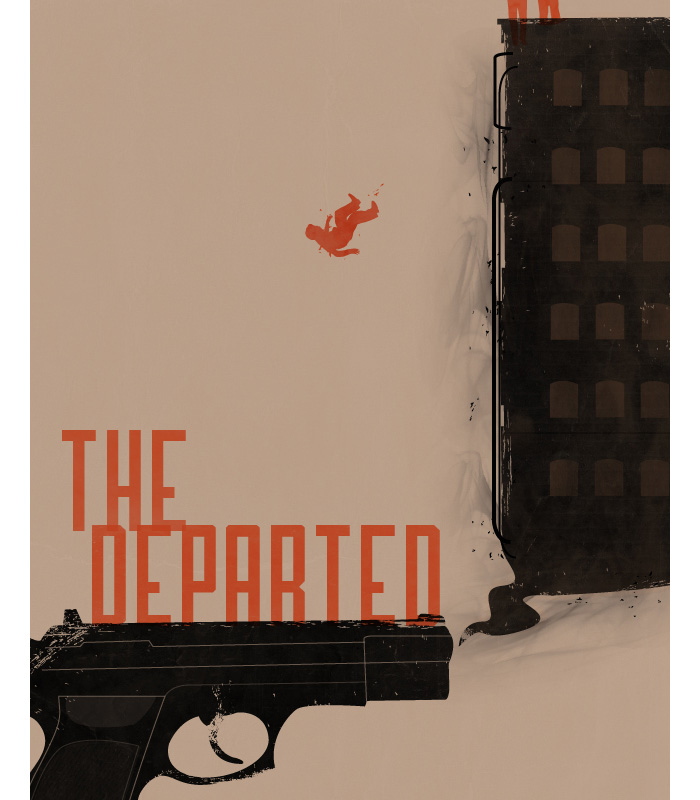The image is a detailed movie poster for "The Departed." Dominating the bottom left corner, a clip art of a black handgun points to the right, with the title "THE DEPARTED" resting on top of it in bold, orange, all-caps text. To the right of the gun, a tall black building rises, vertically striped with rows of lighter brown windows, giving it a distinct look. Emphasizing the sense of peril, an orange silhouette of a man is depicted falling backwards off the building, his arms and legs flailing helplessly as if trying to prevent his inevitable descent. His tie flutters upwards, adding to the dramatic effect. The light tan background contrasts sharply with these dark and bright elements, highlighting the tension and drama of the scene. In the background, near the top of the building, there are hints of other figures, perhaps other individuals on the verge of a similar fate. Overall, the composition evokes a sense of suspense and impending doom.